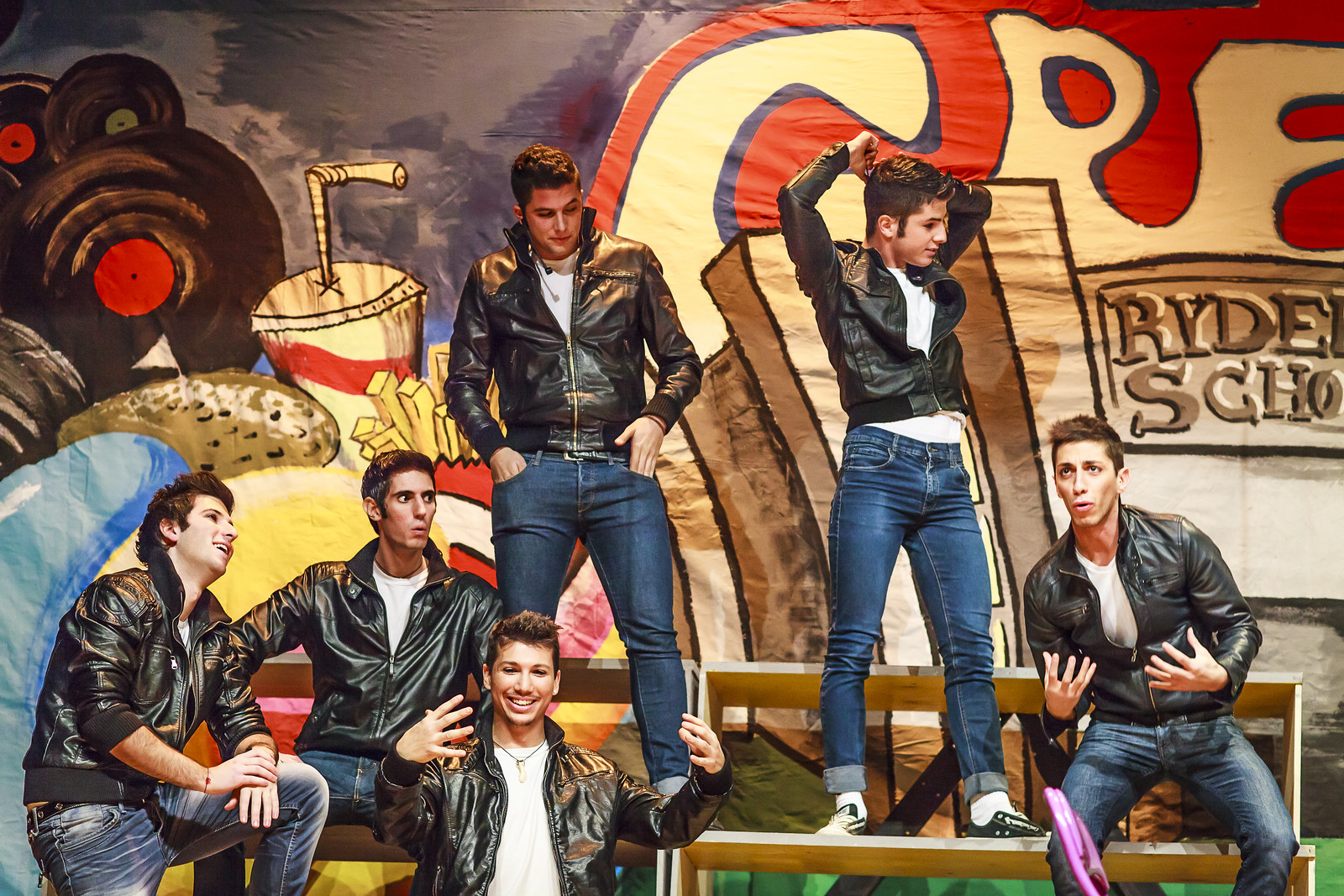The image captures a local production of the famous musical Grease, where a group of six teenage boys are depicted in a quintessential '50s greaser style. All dressed in black leather jackets, white shirts, and blue jeans, they embody the iconic characters of the era. The backdrop is a painted set that partially spells out "Grease" with G-R-E visible, and the stage is adorned with nostalgic elements like vinyl records with colored centers—red and green—scattered around. The boys are positioned on tiered bleachers, giving it a stadium seating feel. The scene is dynamic; one boy stands with his hands outstretched, actively speaking to the group, while another has his hands above his head, and yet another keeps his hands in his pockets. The remaining boys are engaged, with some laughing and others listening intently. A noticeable detail includes a cup with a lid and a straw in the upper left of the image, adding to the casual, retro vibe of the setting. Overall, the scene beautifully captures the essence of a vibrant and lively stage performance.